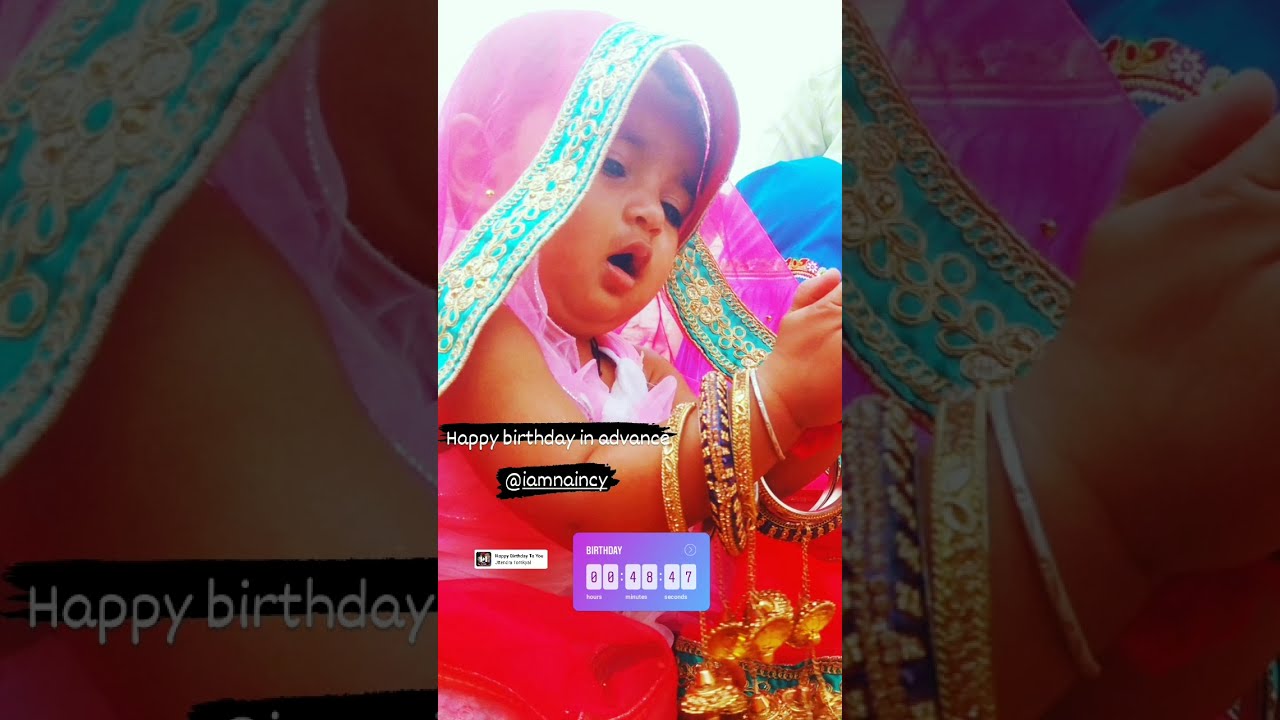The image is a horizontally rectangular photograph with dark strips on both sides, creating a narrowed focus on the vibrant center. The central, vertically aligned portion shows a young, dark-complexioned child clad in bright red clothes, with a pink scarf adorned with blue and gold embroidery framing her face. The child's dark eyes and hair stand out vividly, as does the intricate traditional Hindi attire. Numerous golden and blue bangles adorn her small wrists, complemented by more jewelry possibly belonging to a motherly figure whose arm encircles the child. Text in white lettering on the darkened left section reads "Happy Birthday in Advance @IAMNANCY," while the lower right corner features a purple box with "BIRTHDAY" in uppercase white letters and a running countdown timer below. The overall style blends portrait photography with a zoomed-out, darkened background of the same image to offer a contrast against the detailed, brightly lit center.